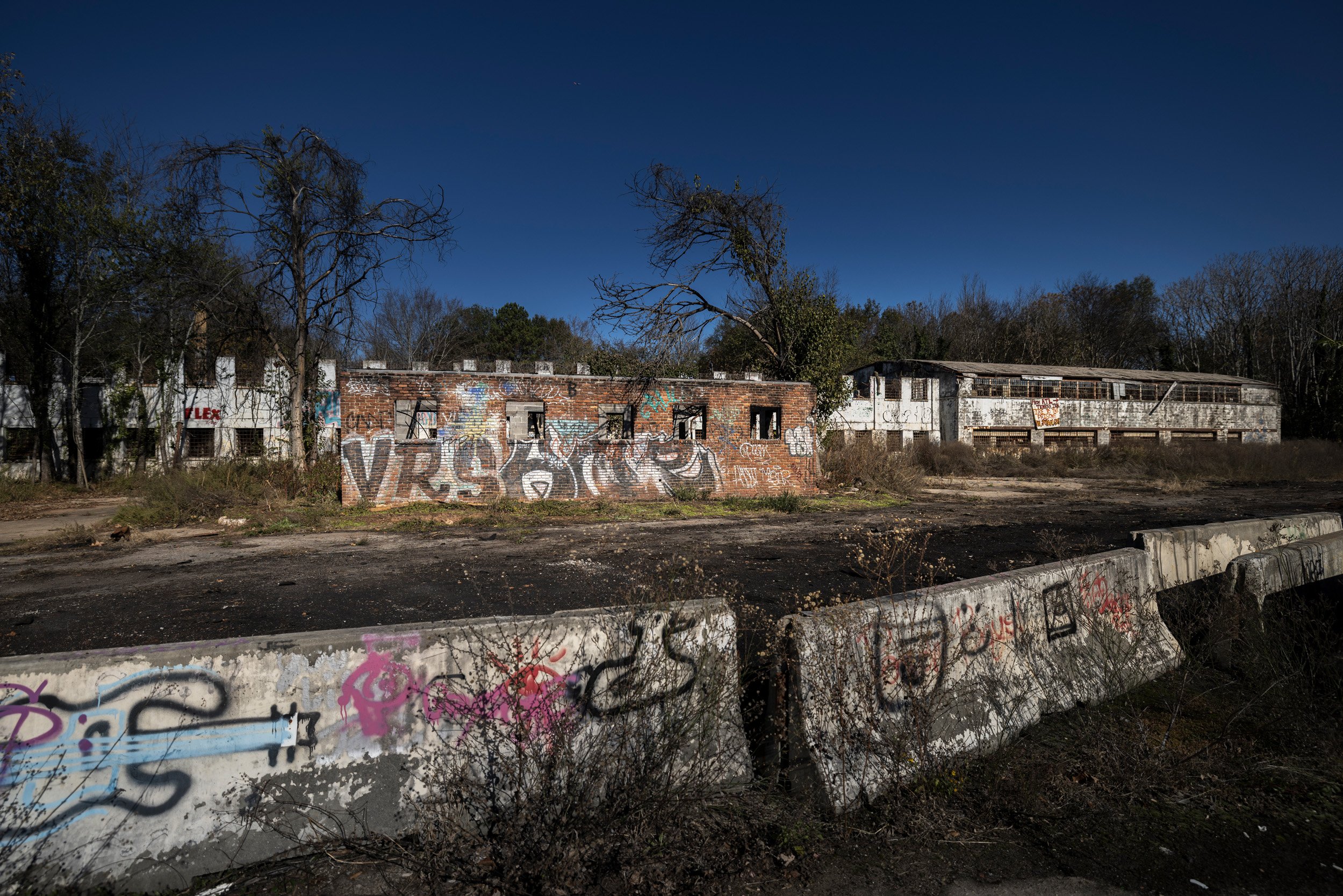The full-color photograph, likely taken around dusk, depicts a desolate and rundown urban area under a very dark blue sky. The scene is filled with trees that are mostly bare, suggesting it is fall. In the foreground, several segmented concrete road dividers are evident, each covered with layers of vibrant graffiti. A patchy dirt road runs through the middle, flanked by unmaintained small bushes and more skeletal trees. Amid these elements, various abandoned buildings stand out, predominately featuring graffiti-splattered exteriors. A prominent, long, white building dominates the background with broken windows and an open roof, giving it a barn-like appearance. On the far left of the image, another white building bears a sign with the letters "K-L-E-X." Additionally, a random brick wall adorned with graffiti, including black block letters outlined in white, disrupts a patch of grass and dirt. The overall feeling conveyed by the image is one of neglect and decay, amplified by the pervasive graffiti and the abandoned ambiance of the area.